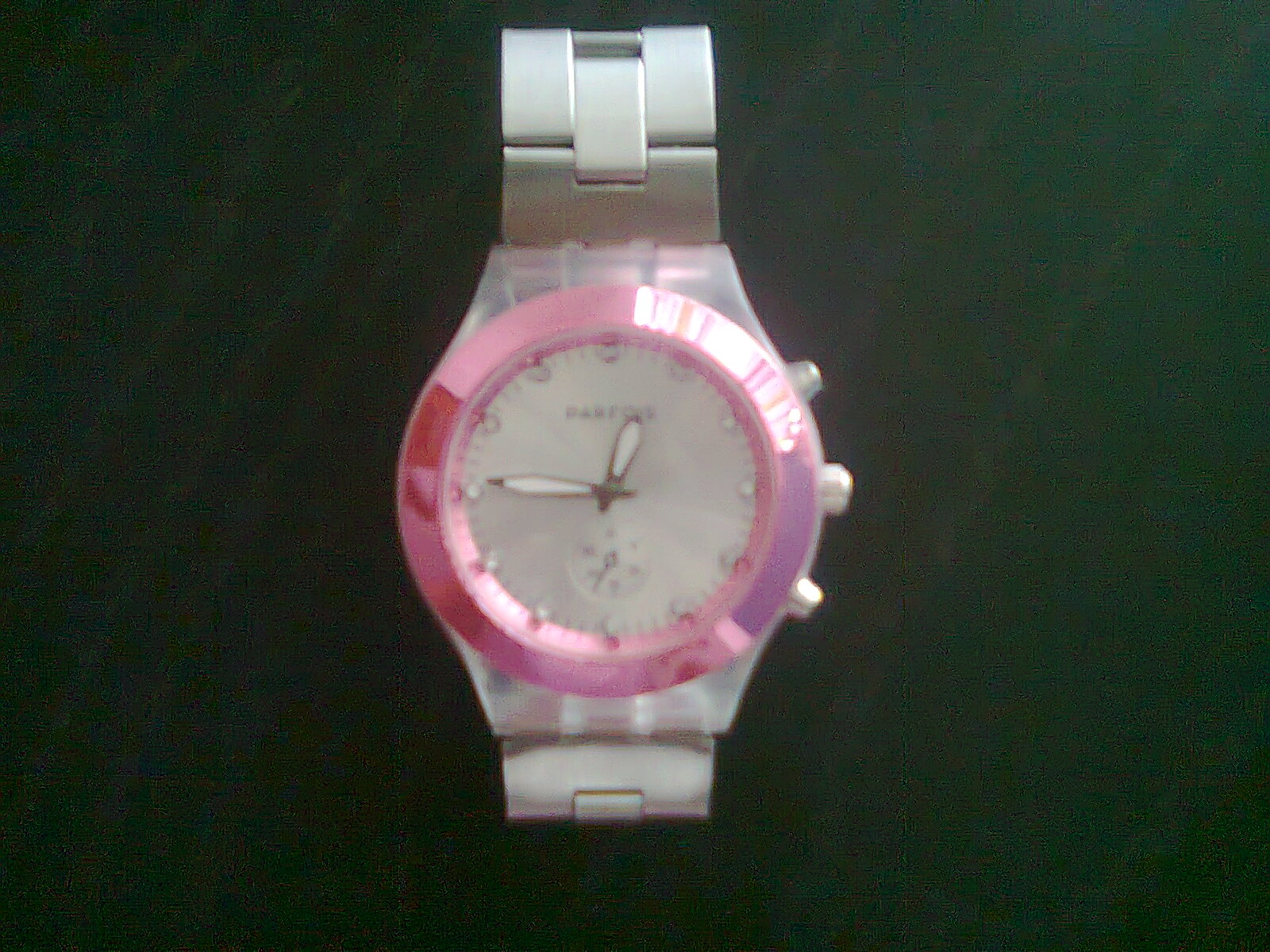This photograph features an elegant wristwatch with a predominantly silver color scheme. The watch boasts a sophisticated silver metal band, adding a touch of sleekness and durability. Encircling the watch face is a striking pink metallic bezel, providing a tasteful contrast. The watch face itself is pristine white, with individual gems set in place of traditional numbers, adding a hint of luxury. The time is indicated by two elongated, teardrop-shaped hands—one larger and one smaller—both white with a fine black border for enhanced readability. Additionally, there are several small adjustment dials on the side for fine-tuning the time and settings. The entire piece is set against a black background, which serves to highlight the intricate details and stunning design of the wristwatch.